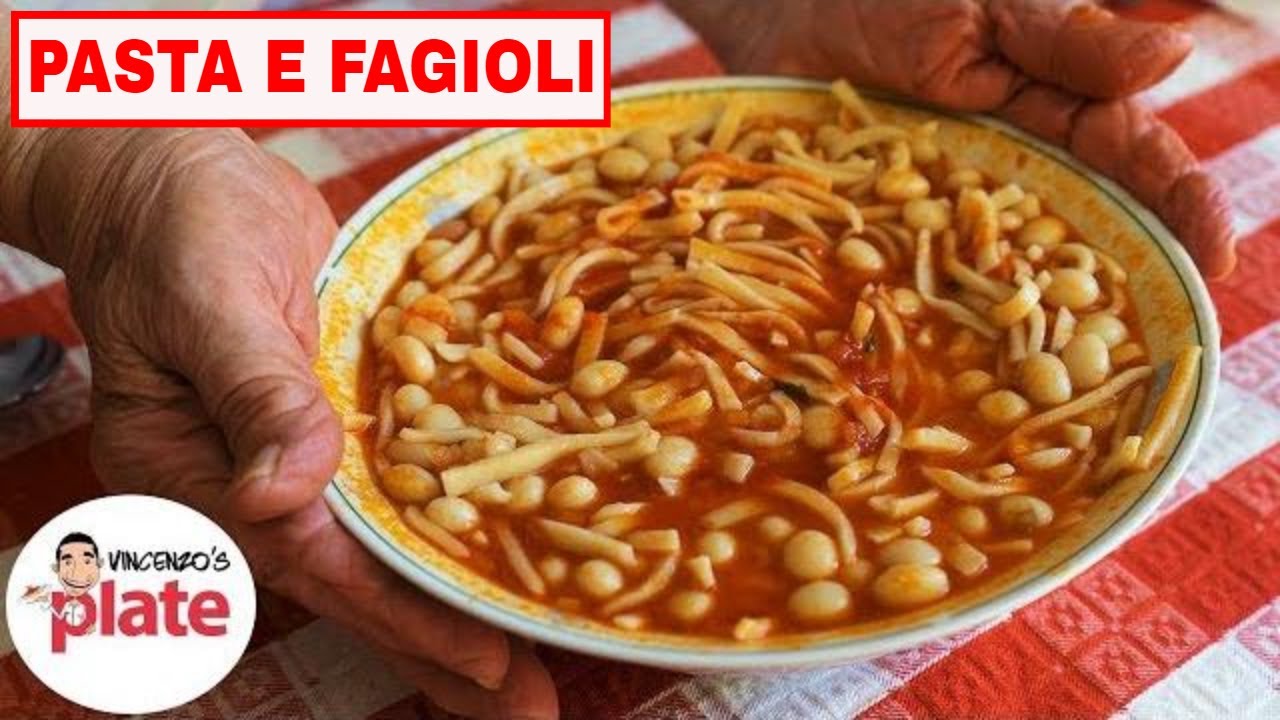The image depicts an advertisement featuring a bowl of soup, prominently displayed at the center. The bowl is white with a thin dark green stripe along its rim, and it is being held by two hands that appear to belong to an older individual, characterized by their wrinkles and slight puffiness. The soup within the bowl has a rich red broth, and is filled with light brown beans and long, thin noodles, similar to spaghetti, with some of the soup splattered against the bowl's edge. This is set against a checkered red and white tablecloth, likely made of plastic or paper. 

In the top left-hand corner of the image is a white rectangle with a red border, containing the text "PASTA E FAGIOLI" in large, uppercase, red block letters. The lower left-hand corner features a circular logo for Vincenzo's, with the text "Vincenzo's" in black and "Plate" in red. Accompanying the logo is a cartoon image of a chef holding a bowl of pasta, emerging partly from the design.